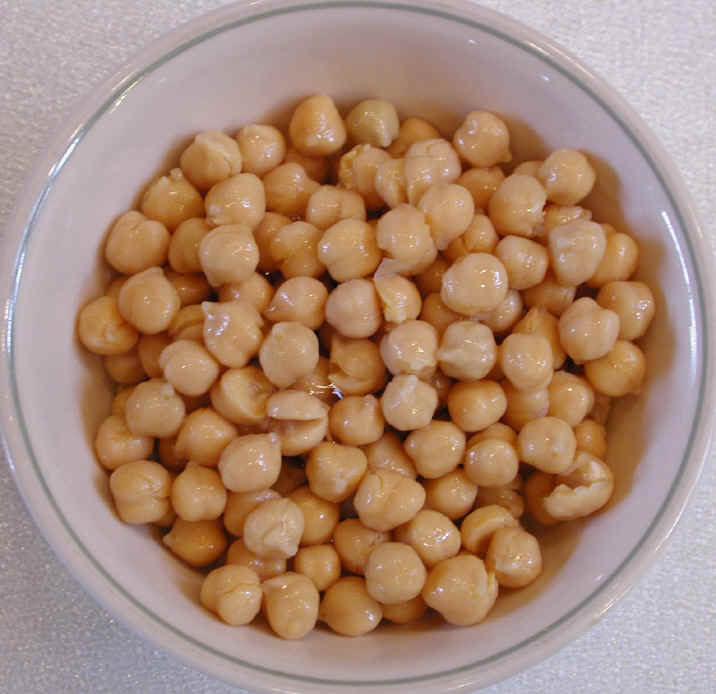This image features a white porcelain bowl, accentuated with a grayish-blue band circling its rim, filled halfway with glossy, wet chickpeas (also known as garbanzo beans or chana). The chickpeas display a light tan to slightly yellowish hue, typical of their natural color, and some appear split open revealing a mushy interior. This suggests they have been boiled, possibly a bit too vigorously judging by the splits. Their shiny appearance indicates they might be coated with a film of water or oil. The bowl is set against a bright white background, possibly a table that has a bumpy texture resembling styrofoam. The scene is brightly illuminated, casting a clear, diffused light over the bowl and its contents, enhancing the glossy surface of the chickpeas.